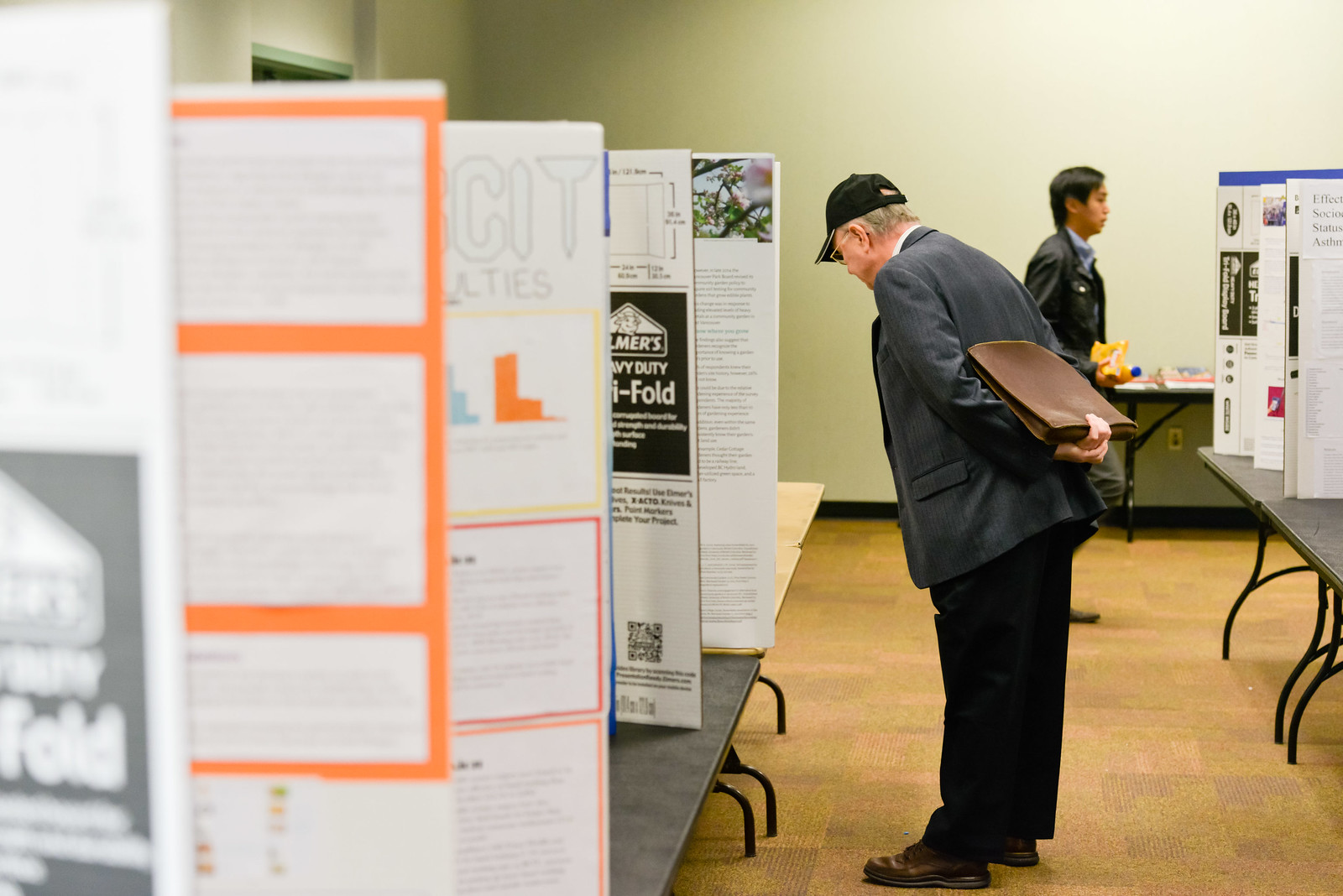The image depicts a bustling science fair set up in a small auditorium or conference room. Several long tables, positioned almost perpendicular to the camera's point of view, are lined up along the walls. Each table holds multiple trifold cardboard displays, showcasing various science experiments and projects. The room is well-lit and features green walls with a brownish-beige and green carpet on the floor. 

In the foreground, an older man, dressed in a gray suit jacket, black pants, and a black baseball cap, is leaning forward to read one of the displays. He wears glasses and holds a brown briefcase behind his back. In the background, a young Asian man is visible, also clad in a suit and carrying a yellow item, as he stands near another display. This detailed snapshot captures the investigative and educational atmosphere typical of a high school science fair.